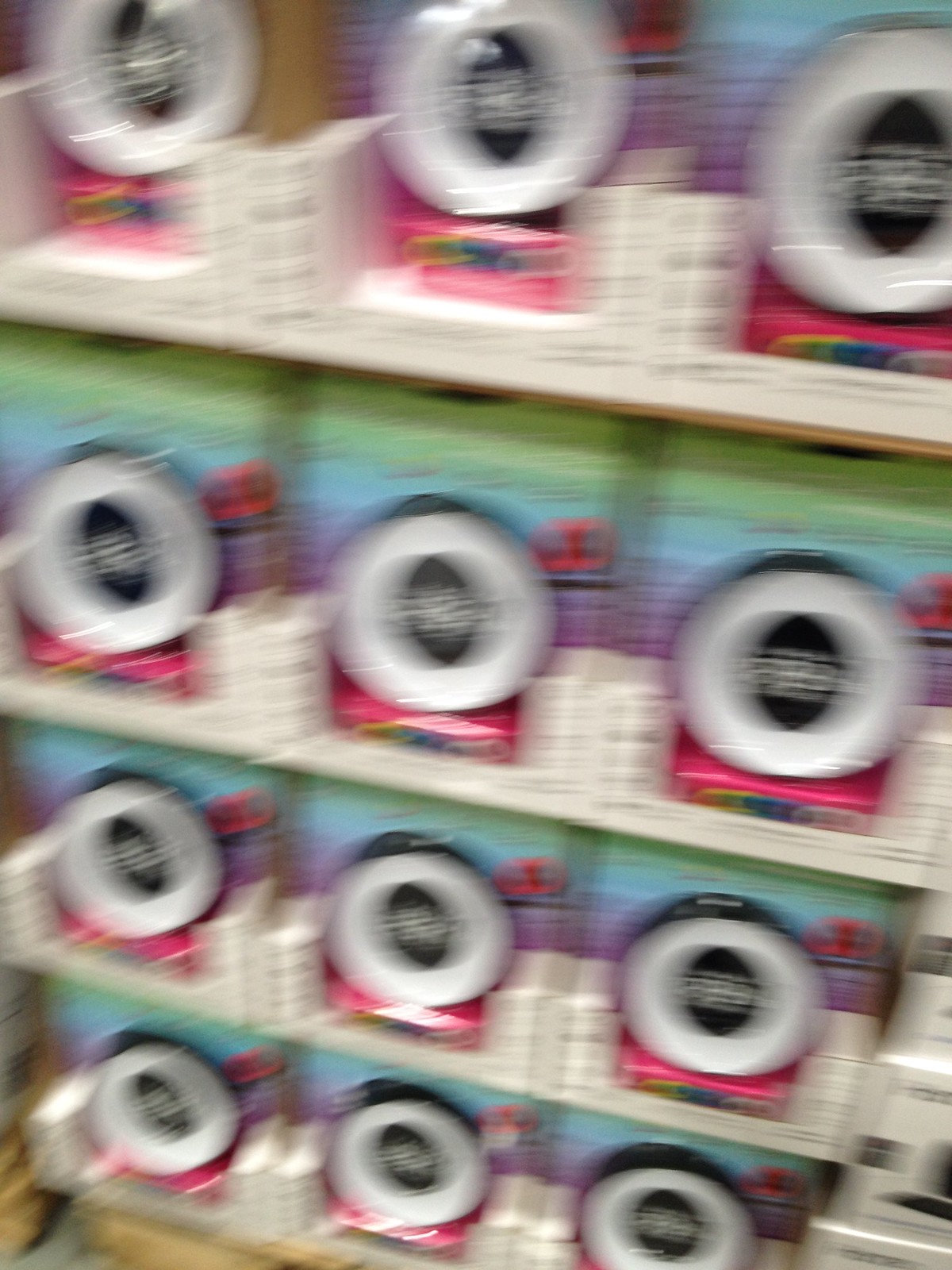The image depicts a retail display featuring four vertical rows of neatly stacked, packaged objects, totaling 12 boxes. Each package is contained within a white box and features a colorful gradient design, beginning with green at the top, transitioning through light blue and purple, and ending with pink at the bottom. Prominently displayed in the center of each package is a white ring with a black interior, while the tops of the boxes are black. The overall setting appears to be a store, as the packages seem to be arranged for sale. The bottom section of the image shows a light brown surface, possibly a pallet, on which the boxes are arranged. The image is slightly blurry, adding a subtle vintage effect to the scene.